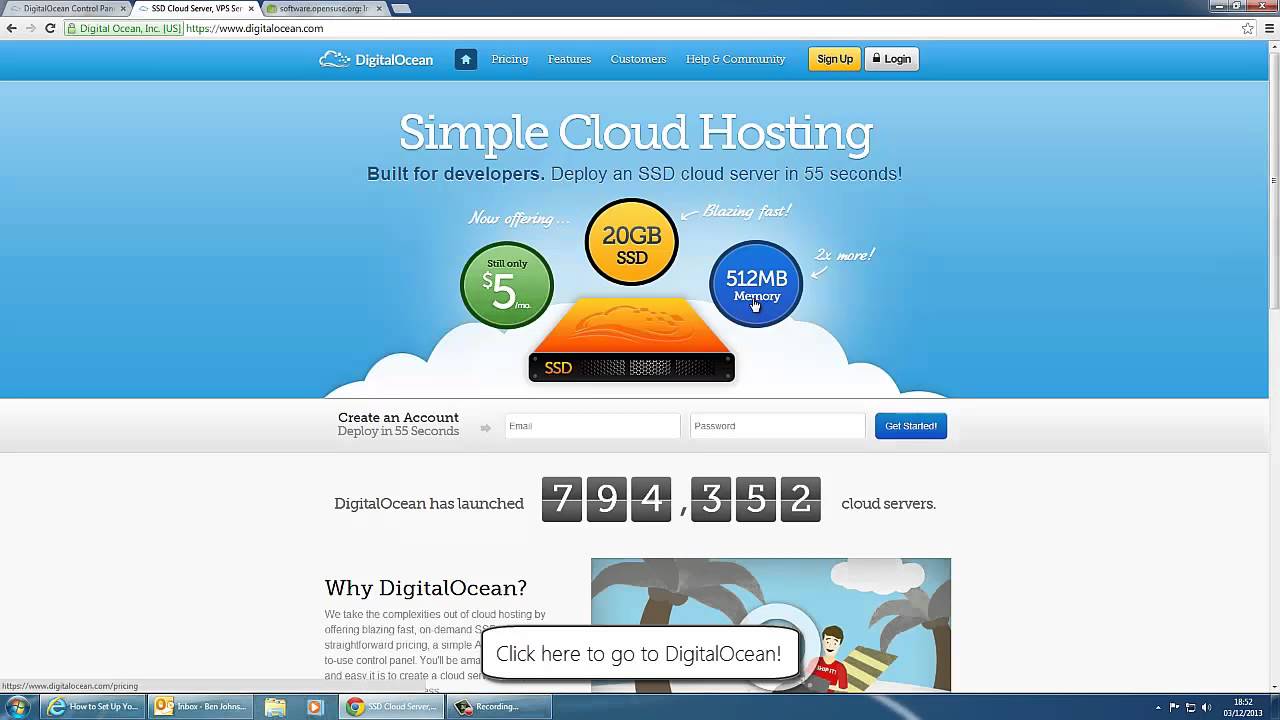This screenshot from the digitalocean.com website features their official emblem resembling watery clouds at the top left corner. To the right of the emblem, the navigation menu includes buttons labeled 'Home', 'Pricing', 'Features', 'Customers', 'Help', and 'Community'. Next to these, there are two buttons: a yellow 'Sign Up' button and a gray 'Login' button.

The main section of the page showcases the headline "Simple Cloud Hosting" with a subheading "Built for developers deploy an SSD cloud server in 55 seconds." Below this, a promotional text reads "Now offering..." followed by details within various color-coded circles: a green circle with "Still only $5 a month," an orange circle with "20 GB SSD," and a blue circle with "512 MBs memory." Notably, the cursor appears as a pointing finger over the "512 MBs memory" circle, emphasizing key information.

Additional text highlights "Blazing fast two times more memory." Further down the page, there is a clickable bar labeled "Click here to go to DigitalOcean," leading to more details. A paragraph beneath it elaborates on the advantages of choosing DigitalOcean.

This detailed layout captures the essence of the website's offerings and navigation for potential users.